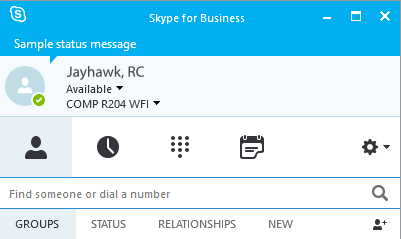The image appears to be a screenshot of a Skype for Business interface captured from a cell phone. The top portion of the screen features a blue bar with "Skype for Business" prominently displayed in white text at the center. On the upper left corner of this blue bar, there's an icon resembling an oval shape with an 'S' in the center.

Beneath this section, there is a status message reading "Sample status message." To the left, users can see a gray circle with a white person icon inside, accompanied by a green checkmark indicating availability. Next to this icon, the text reads "Jayhawk RC available. Comp R2 R2O4 Wi-Fi."

Below this information, a blue-highlighted button shows that someone has selected the person icon. Adjacent to this button, there are several symbols: a clock, a dotted down arrow, a document-like icon, and a tool symbol resembling a bolt.

A search bar is positioned underneath these icons, containing the placeholder text "Find someone or dial a number" and a magnifying glass icon on the right side of the bar.

Further down, there is a blue-highlighted selection on "Groups," next to options labeled "Status," "Relationships," and "New." In the bottom right corner of the screen, a small black person icon is visible.